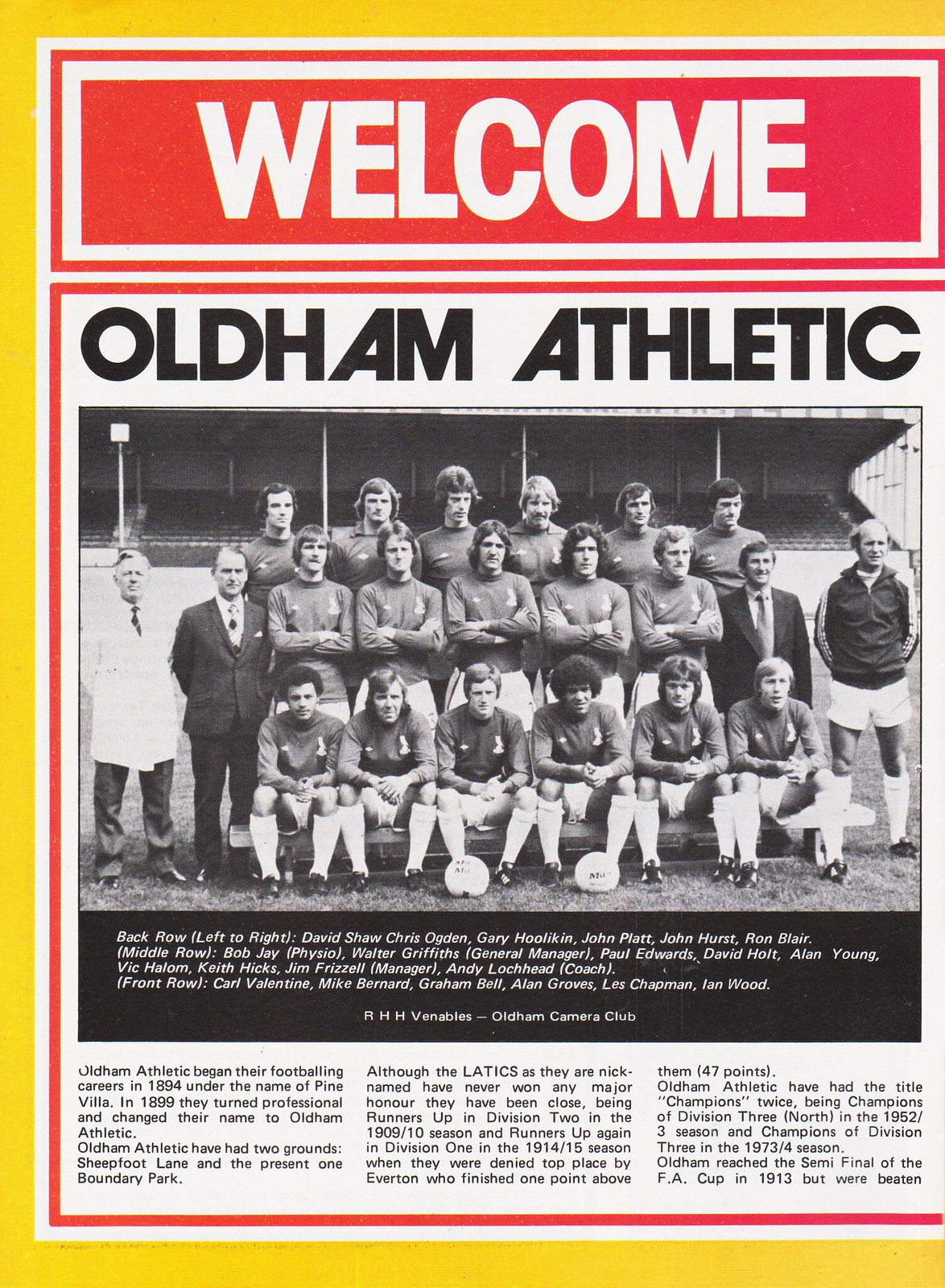The top of this magazine or newspaper article is set against a vibrant red background, prominently featuring bold, all-capital white text that reads "WELCOME." Just below this welcoming statement, in similarly bold, all-capital black letters, the name "OLDHAM ATHLETIC" commands attention. Centered on the page is a striking team photo: two orderly rows of players, the back row standing with their arms confidently crossed, while the front row sits in classic, white socks. Beneath this team image, the article is presented in three neatly arranged, vertical columns of text. The entire article is framed by a thin red line, adding to its visual appeal, and a half-inch from the edge, a distinctive yellow border completes the design.